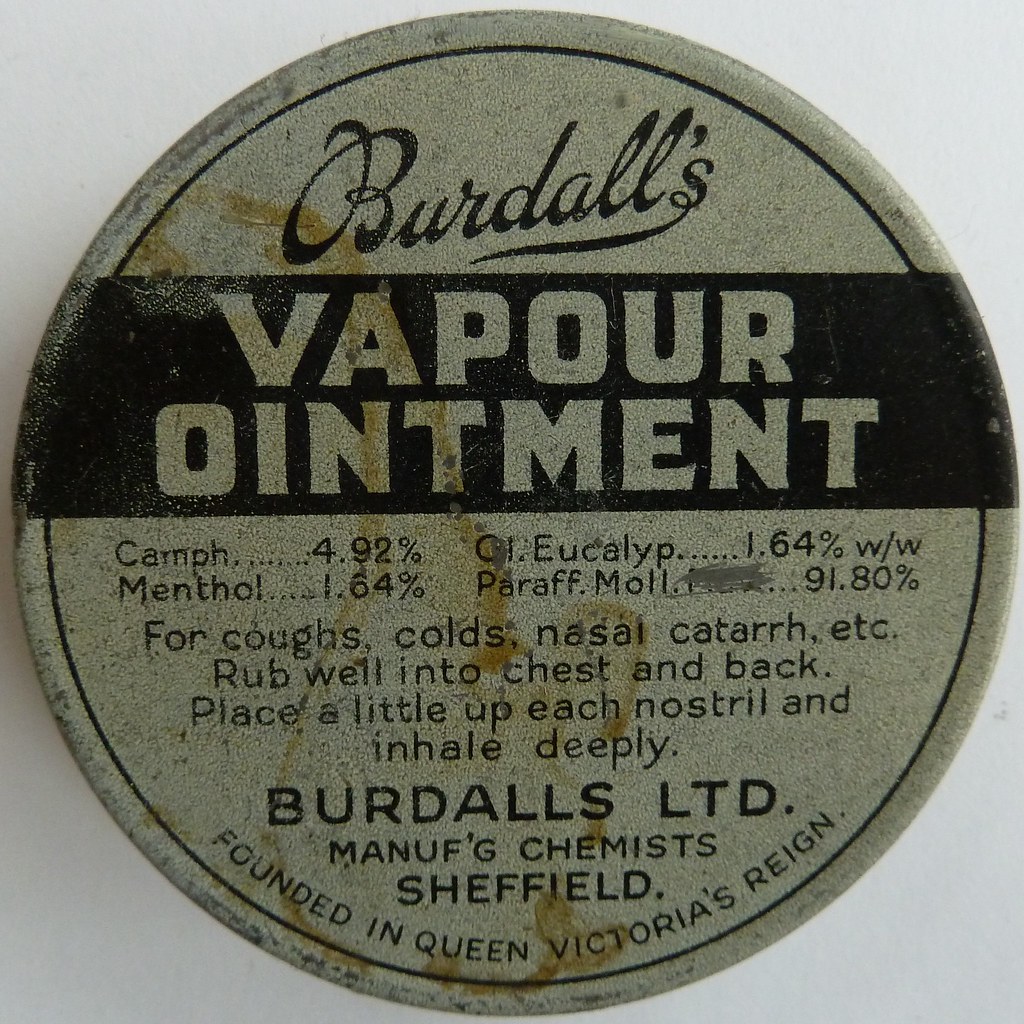The image depicts a circular, gray tin of Burdolls vapor ointment resting on a white surface. The tin is outlined by a black border, and the cap is old and rusty with visible blurs and patches of dirt. At the top of the can, "Burdolls" is prominently displayed, with the "S" underlined and curving up to the "R." Below this, a black ribbon banner with gray letters reads "Vapor Ointment." Beneath the ribbon, the composition of the ointment is listed as: Karmf 4.92%, Menthol 1.64%, Oiglip 1.64%, W/W, and Paraf Myl (partially scratched out) 91.80%. Further down, the directions for use are printed: "For coughs, colds, nasal catarrh, etc., rub well into chest and back, place a little up each nostril and inhale deeply." At the bottom of the can, the text reads: "Burdolls Limited, Manufacturing Chemists, Sheffield, founded in Queen Victoria's reign." The can also has a brownish-colored stain towards the left and middle, reinforcing its aged and worn appearance. The background of the image is gray, blending slightly with the worn gray tones of the tin itself.